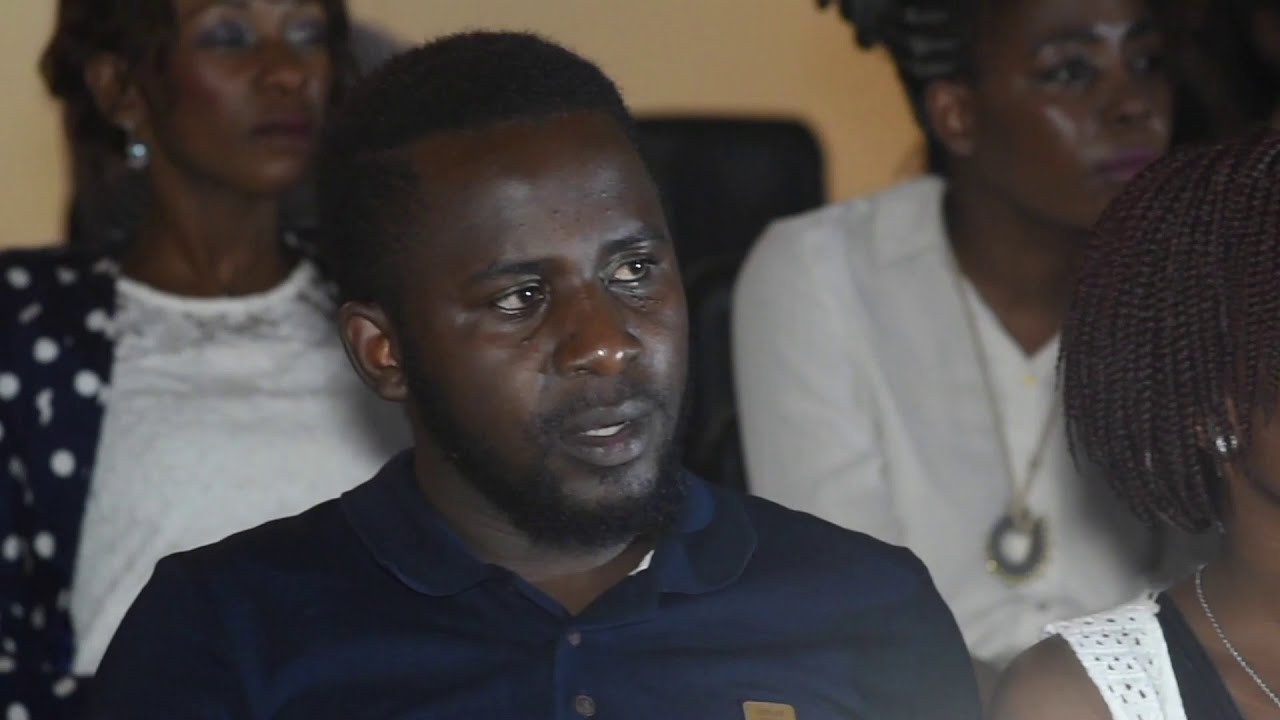The image captures a serious and contemplative scene featuring four individuals who appear to be part of an audience, possibly in a professional or formal setting. All individuals have dark skin and are facing the front, but their gazes are directed towards the right side of the image. 

Prominently in the foreground, at the center, sits a man in his late 20s or 30s, with short black hair and facial hair, wearing a navy blue collared short-sleeved polo shirt, buttoned up with one button left open. His expression is serious yet not overly stern.

To his right, a woman can be partially seen; she has short braids and is dressed in a white sleeveless shirt. Only parts of her hair, leg, and shoulder are visible, along with her necklace and earrings.

Behind the man, slightly to his left, is a woman wearing a black coat adorned with white polka dots. Her hair is up, and she has earrings that add to her business-casual attire. Next to her is another woman, clad in a gray suit, with her hair braided and styled up, also wearing a necklace.

The backdrop of the image is light brown, contributing to a neutral, serious atmosphere which suggests the setting could be a classroom, meeting, or formal gathering. The overall coloration in the photograph includes various shades of brown, black, white, blue, and a hint of silver and pink, adding to the richness and detail of the scene.